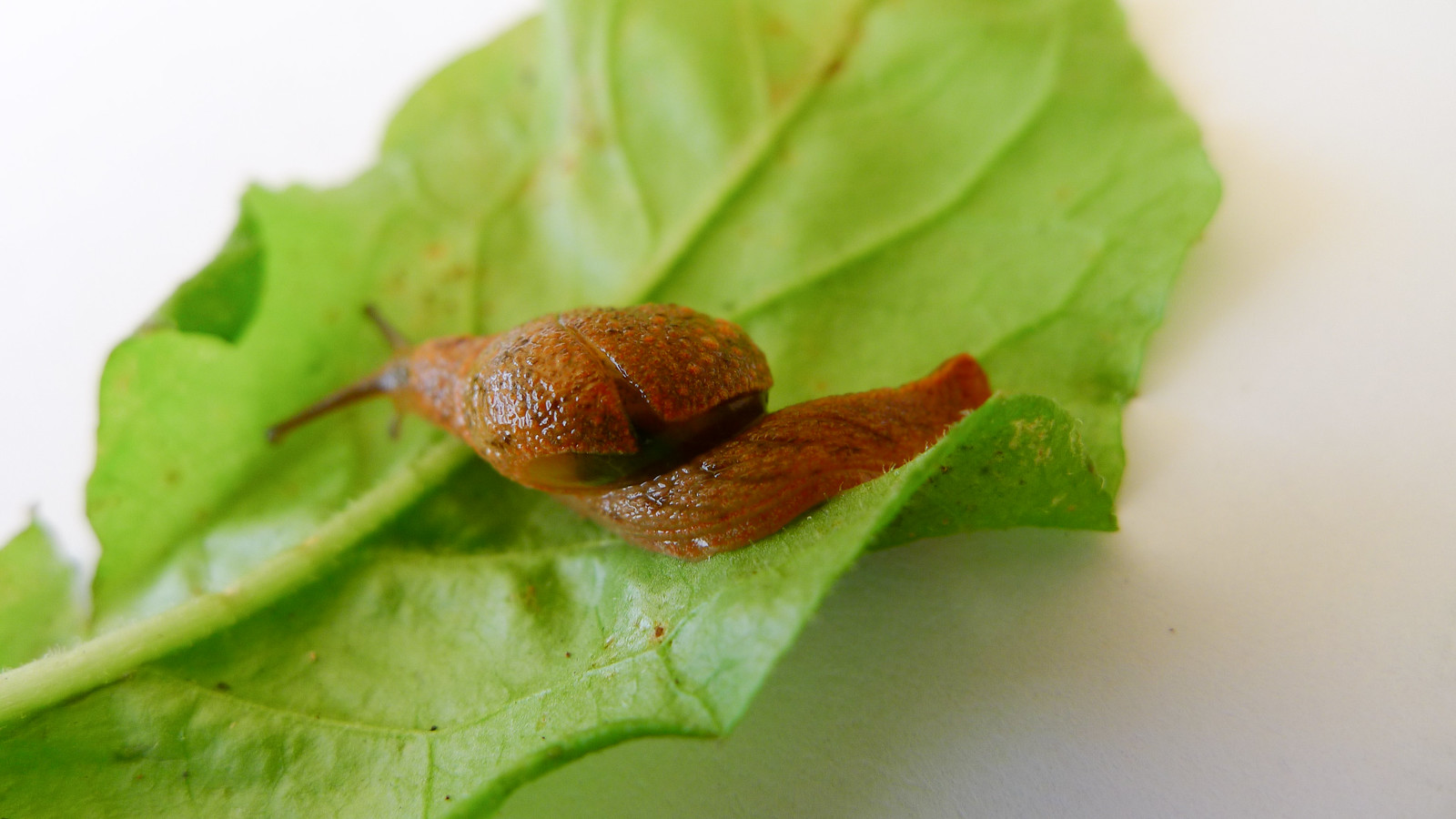This detailed color photograph captures a close-up of a reddish-brown slug positioned slightly left of center on a large green leaf. The slug's body exhibits a reddish hue with dark brown stripes, especially prominent on its tail. The slug's skin has some lighter brown bumps giving it a textured appearance. The head, facing away from the camera, features two dark brown antennae extending forward as if it were seeking its path. The slug's body thickens toward its rear, which extends to the right and ends in a tail-like tip that veers off slightly. The green leaf it rests on has a pronounced central vein with smaller veins branching off. The leaf, appearing slightly wilted, casts a shadow on an otherwise stark white background, accentuating the slug and the leaf's intricate details.